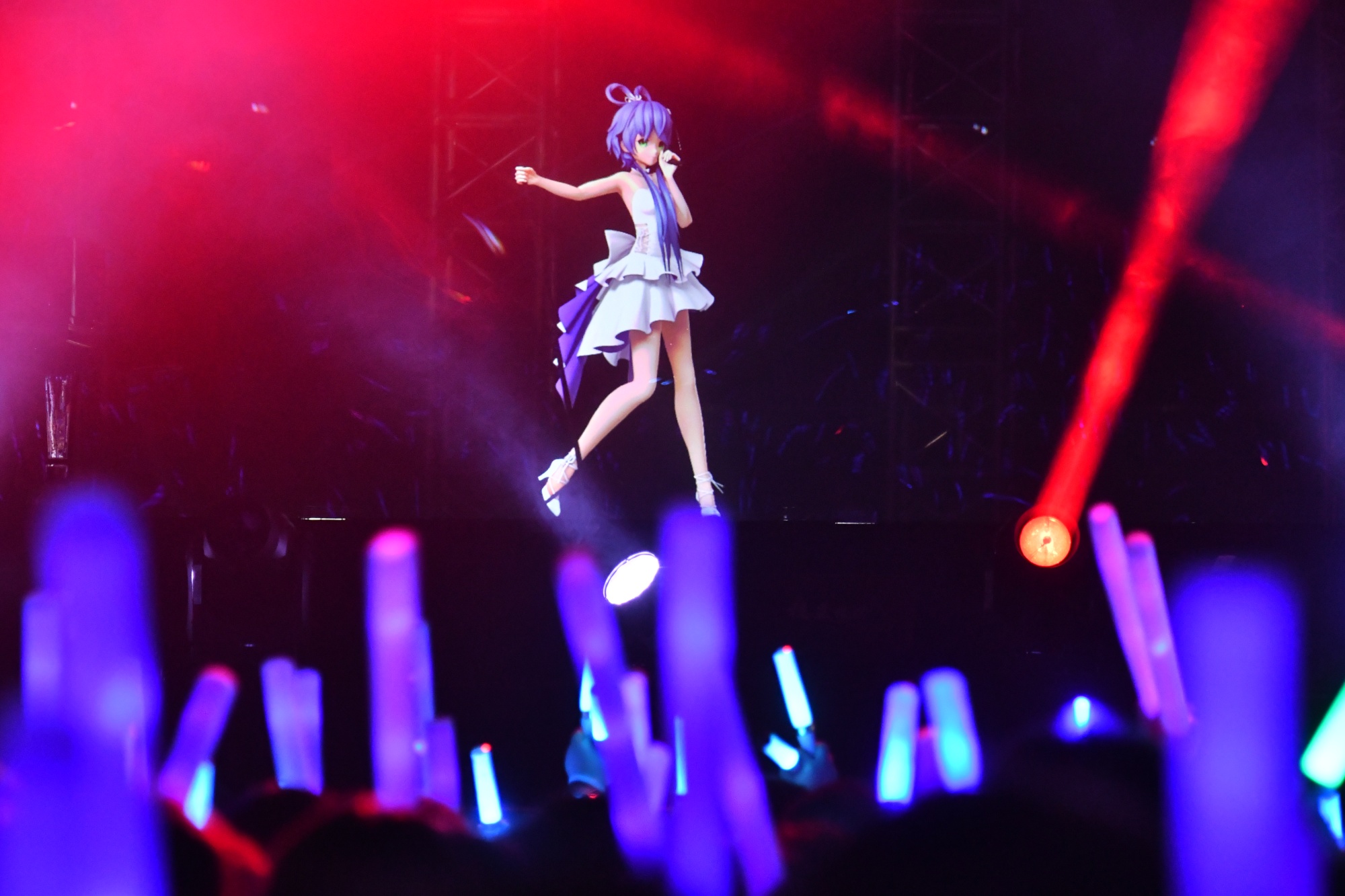This image appears to be a screenshot from a cartoon or video game, depicting an animated anime girl performing on a stage. The setting evokes a concert atmosphere, with a wide vertical composition featuring a dark background illuminated by vibrant red and purple lights streaming from the top left and right corners. The girl, with light purple hair styled either in short pigtails or with a scarf, stands confidently singing into a microphone held in one hand while the other arm is extended at shoulder height. She dons a sleeveless white dress with a ruffled skirt that reaches her knees, accentuated by a black or purple ruffle hanging from the back, and white high-heeled shoes.

She is facing slightly towards the right side of the image and positioned as if dancing, adding dynamic movement to the scene. The perspective is from the crowd, looking up towards the stage, capturing the animated energy of the performance. The audience members are holding glowing purple cylinders, simulating concert glow sticks, which enhance the lively concert vibe. In the background, beyond the stage and the performer, a mass of additional glowing cylinders and indistinct heads suggests a larger crowd, also immersed in the concert experience.